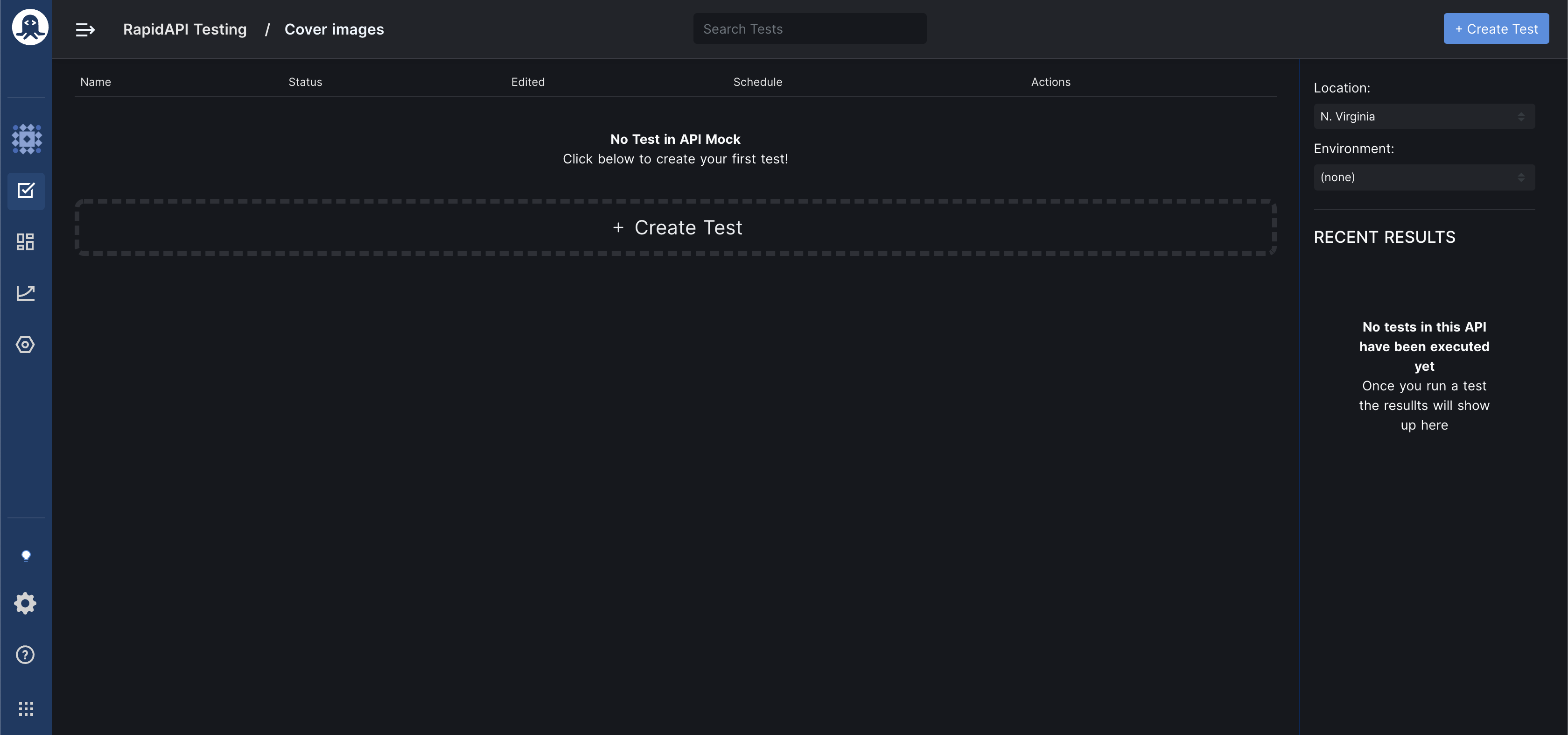The image appears to be a screenshot of a web page featuring a user interface for rapid API testing. The background is predominantly a dark grayish-black color, almost black, with a thin vertical strip in navy blue on the left-hand side. At the top of this strip, there is a circular logo of a confused squid whose eyes are depicted as left and right arrows, and its arms are extended outward in a nonplussed manner.

This navy blue sidebar contains several logos:
1. A set of geometric shapes
2. A square with a checkmark inside
3. Various rectangles
4. A graph-like icon
5. A hexagon with a circle inside

At the bottom of the sidebar, there are icons for a light bulb, a gear, a question mark for help, and a three-by-three grid pattern.

In the top right-hand corner of the main section of the page, there is a prominent blue button labeled "Create Test" in white text. Just below this, a slightly lighter gray bar spans the top of the screen, containing the text "Rapid API Testing / Cover Images." This bar includes columns labeled: Name, Status, Edited, Schedule, Actions, and features a search bar labeled "Search Tests."

The main area of the screen displays a message stating, "No tests in API mock. Click below to create your first test." Below this message, there is a long rectangular button with dashed lines around it, labeled "+ Create Test."

On the right-hand side, there is a section titled "Recent Results" which indicates that no tests have been executed in this API yet. A note states that results will appear here once a test has been run.